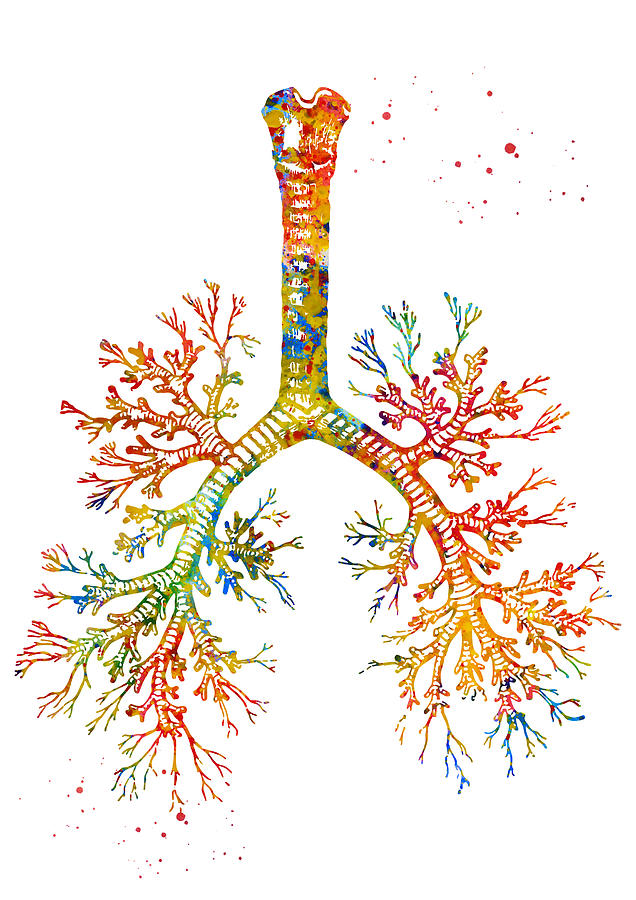This vibrant and intricate painting presents a detailed internal view of the human lungs, highlighting the bronchial tree-like structure against a white background. The central windpipe, depicted in varying shades of red, yellow, and blue, runs vertically and branches off into progressively smaller tubes, reflecting the structure of a tree limb with each branch adorned in an array of colors including red, yellow, green, turquoise, and dark blue. The image bears the artistic touch of paint splatters, with noticeable red specks on the top and bottom corners, emphasizing its hand-painted origin. The shape at the top aligns with the characteristic form of the Adam's apple, further signifying a respiratory anatomy. Overall, the artwork masterfully combines anatomical accuracy with vivid rainbow hues, creating a dynamic visual representation that mirrors both a natural root system and coral structures.